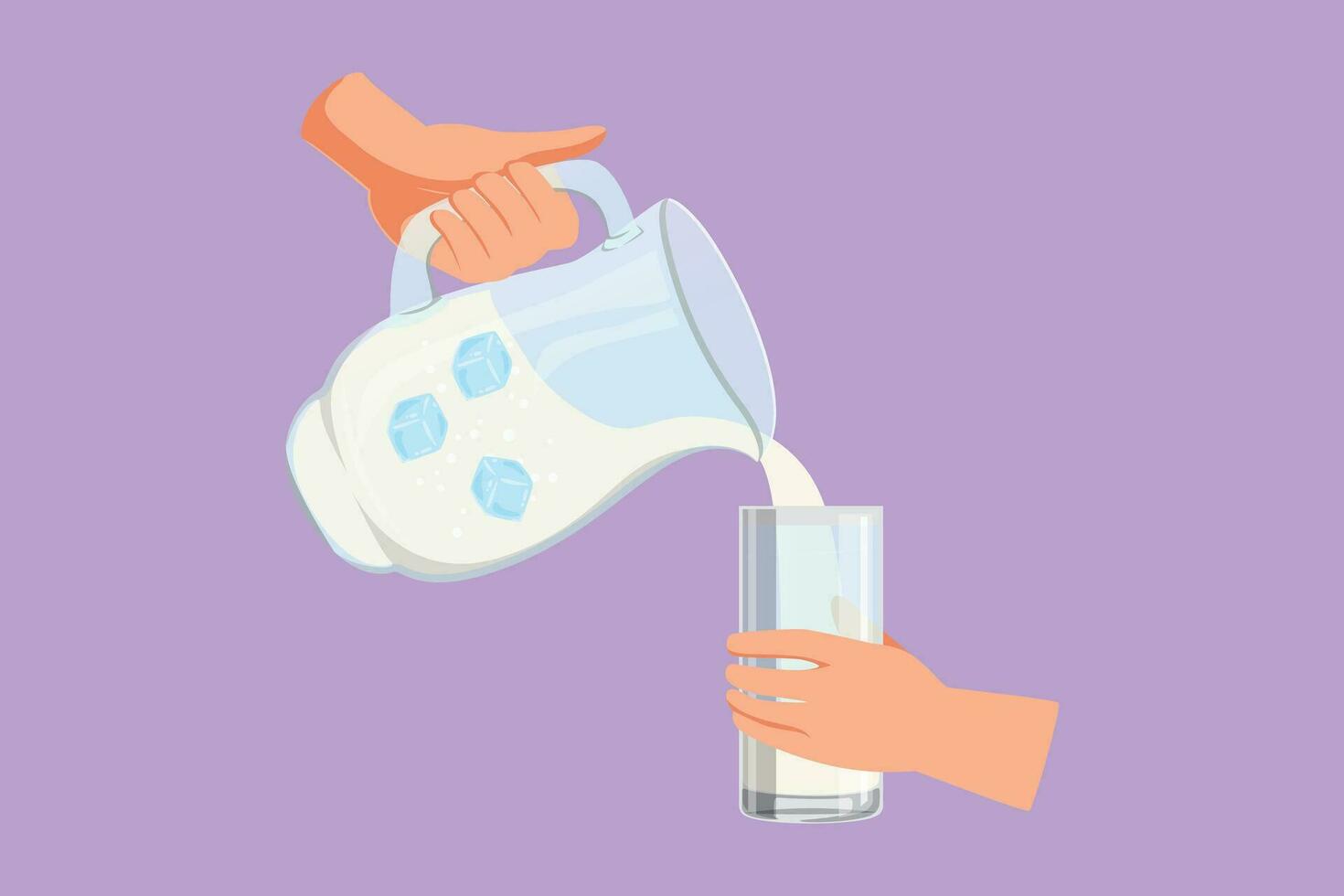The illustration features a simplistic design with a solid violet background. In the foreground, two hands are prominently depicted. The larger hand on the left, which appears to be that of an adult, is holding a clear pitcher made of either glass or plastic. This pitcher contains a whitish liquid with three bluish ice cubes floating inside, and sparkly designs are visible within the liquid, enhancing its visual appeal. The liquid is being poured into a glass held by a smaller hand on the right, likely that of a child. Both hands have a pinkish hue, and the overall composition of the image emphasizes the interaction between the two figures through the act of pouring and receiving the liquid.